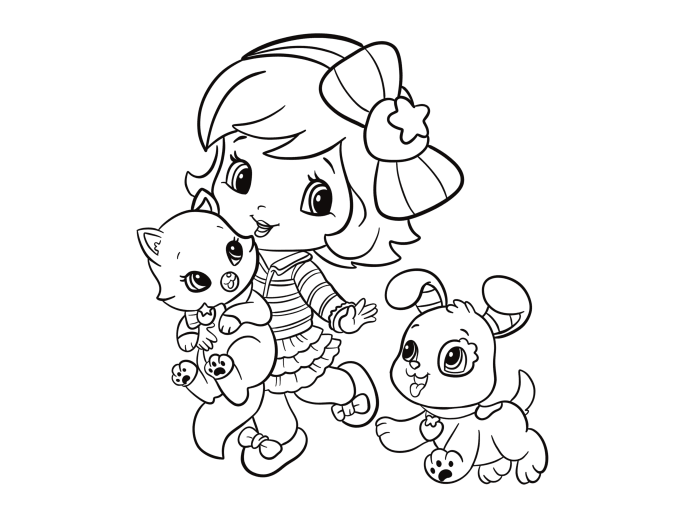This black and white image, reminiscent of a drawing intended for a children's coloring book, features a charming scene of a little girl with a bow in her shoulder-length hair. The girl, positioned on the left side of the image, is holding a kitten with one hand around its chest, while a happy puppy follows closely behind her. Both the girl and the animals have wide, joyful smiles on their faces.

The girl, possibly a toddler, stands out with her expressive wide eyes and is adorned in a striped sweater and a frilled skirt. Her outfit is complemented by small shoes, each decorated with a bow. The kitten in her arms looks up at her affectionately, displaying paw prints on the bottoms of its feet. The playful puppy, marked by a distinctive spot over its left eye, appears to be chasing after them with a strawberry-like collar around its neck.

The scene captures a happy little outing, with the girl, her kitten, and her dog all exuding a sense of joyful companionship as they venture together. The image is left in black and white, inviting colors to be added to bring the wholesome moment to life.